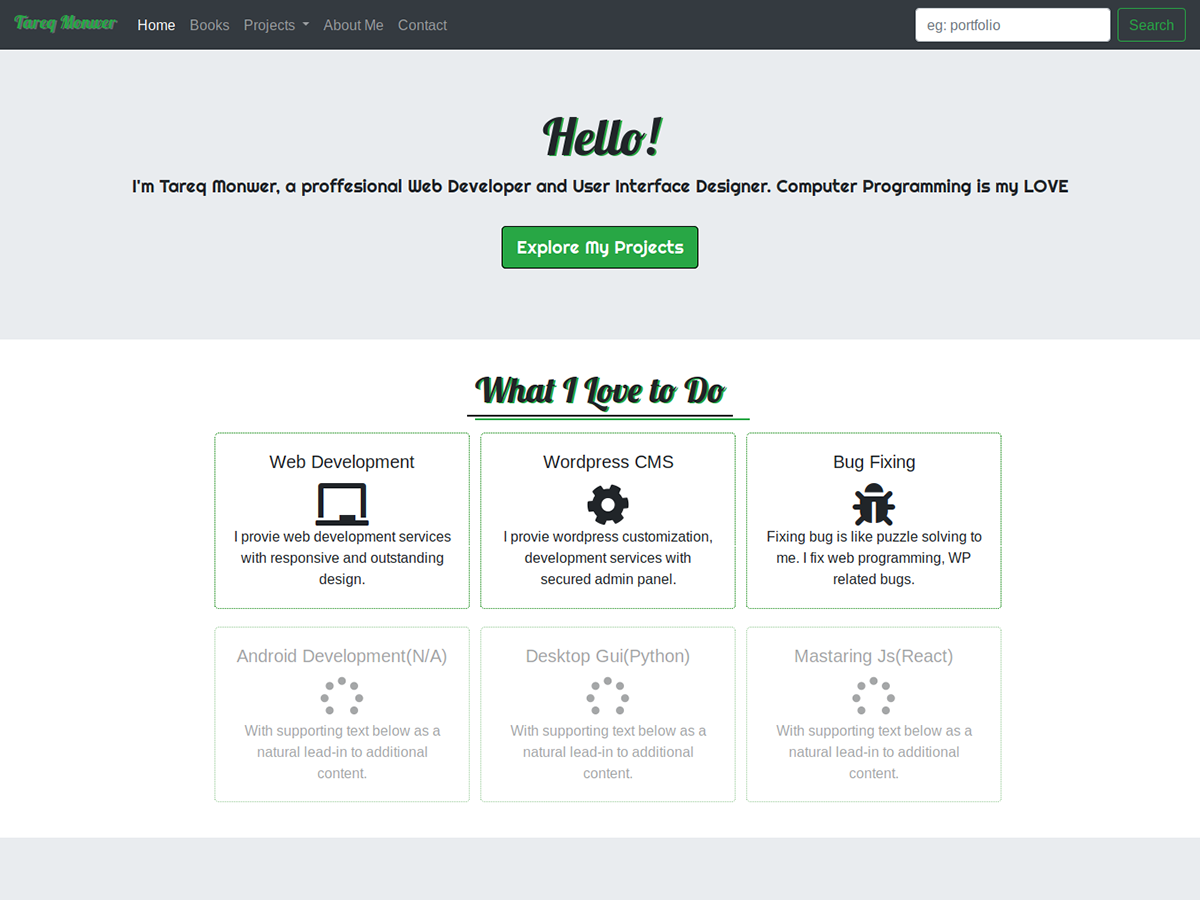In the upper right-hand corner of the image, there is text in green letters that reads "Tareq Monwer," spelled T-A-R-E-Q space M-O-N-W-E-R. To the right of this text are several tabs arranged horizontally, labeled from left to right: Home, Books, Projects, About Me, and Contact. The Home tab is highlighted in white, indicating that it is currently selected, while the other tabs are in gray. 

In the very upper right-hand corner is a search bar with the text "EG-Portfolio" inside it. 

At the top center of the photo, the word "Hello!" is prominently displayed in green letters. Below this, another line reads, "I'm Tareq Monwer, a professional web developer and user interface designer." The line ends with a period. The phrase "Computer programming is my LOVE." appears next, with "LOVE" fully capitalized for emphasis.

Below this introductory text, there is a clickable option that says "Explore My Projects."

Further down, the section titled "What I love to do," also in green letters, introduces six rectangular boxes that provide more details about Tareq Monwer's services and expertise. 

In the first row, from left to right, the boxes are labeled as follows:
1. Web Development: A description reads, "I provide web development services with responsive and outstanding design."
2. WordPress CMS: "I provide WordPress customization development services with a secured admin panel."
3. Bug Fixing: "Fixing bugs is like puzzle solving to me. I fix web programming, WP-related bugs."

In the second row, from left to right, the boxes are labeled:
4. Android Development (M.A.) 
5. Desktop GUI (Python)
6. MasteringJS (React) 

Each of these labels outlines specific areas of expertise and passion, presenting a comprehensive view of Tareq Monwer's professional skills and services.